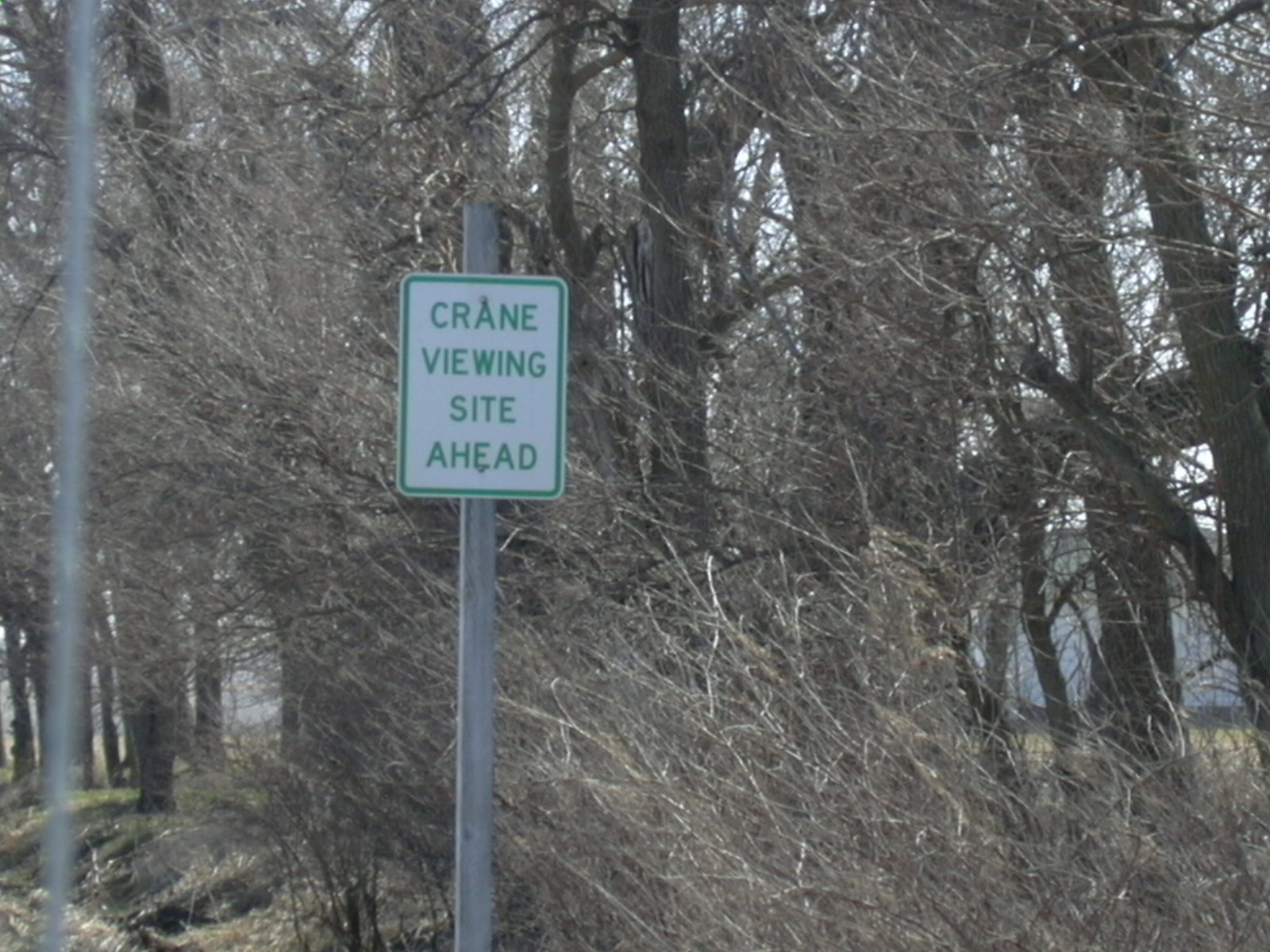A picturesque scene composed of various natural and man-made elements. In the foreground, a silver pole supports a rectangular white sign bordered in green, prominently featuring green text that reads "Crane Viewing Site Ahead." To the far left, a metal pole stands vertically. The ground is primarily covered with dry grass, reflecting the dormant or possibly dead state of the vegetation. Behind the sign, a multitude of dry branches and trees stretch across the middle ground, creating a dense, somewhat barren forest-like backdrop. The sky overhead is a clear and vivid blue, providing a stark contrast to the earthy tones of the landscape below.